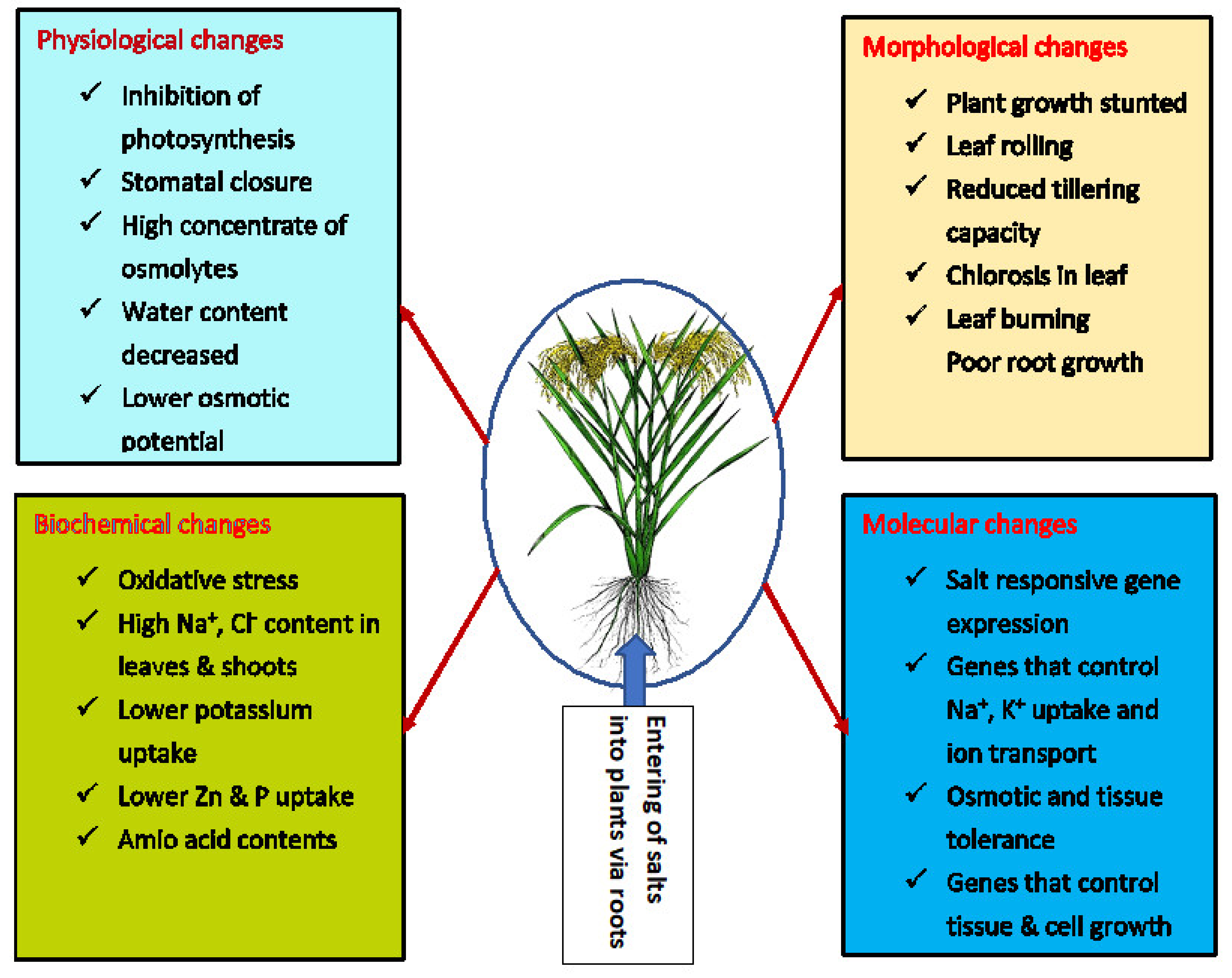This detailed image from a textbook appears to be an explanatory graph showcasing different types of changes plants undergo. Central to the image is an illustration of a yellow-flowering plant with long green spiky leaves and visible roots, all enclosed within a blue oval. The heart of the plant, set against a white background, prominently features a vertical arrow labeled "entering of salts into plants via roots," pointing to the roots.

Surrounding this core graphic, four arrows extend outward toward each corner, each directing towards a distinct text box that elaborates on various changes. The text boxes are as follows:

1. **Upper Left:** A blue text box titled "Physiological Changes" in red text, detailing points such as inhibition of photosynthesis, high concentration of osmolites, water content decrease, and lower osmotic potential.
   
2. **Upper Right:** A blue text box titled "Morphological Changes" in red text, with detailed information underneath.

3. **Lower Left:** A blue text box titled "Biochemical Changes" in red text, accompanied by detailed explanations.

4. **Lower Right:** A blue text box titled "Molecular Changes" in red text, also containing detailed points.

Each description is in black text, while all titles are emphasized in red. The intricate composition of arrows, colors, and structured information provides a comprehensive visual representation of the physiological, morphological, biochemical, and molecular changes in plants.